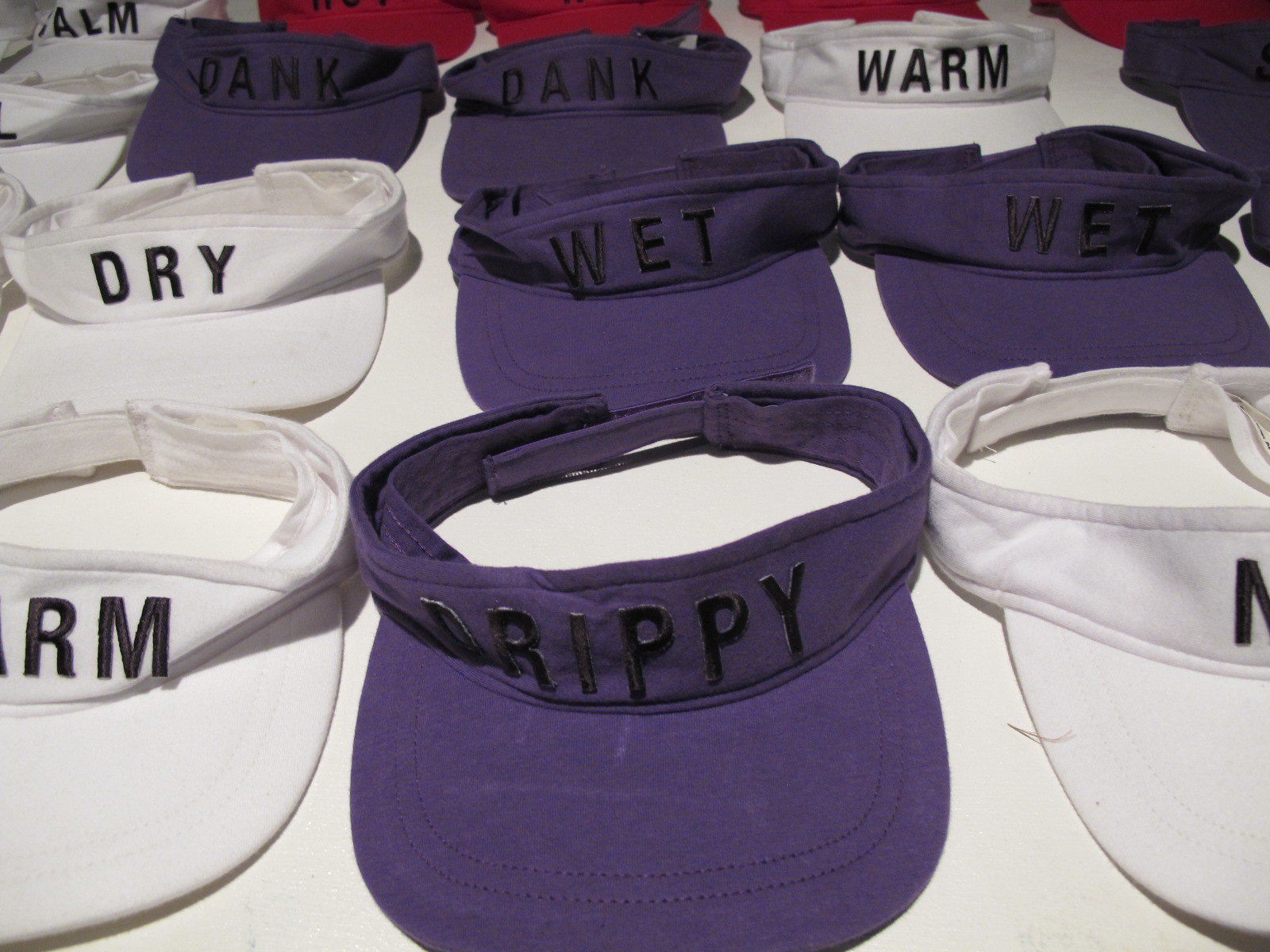The image features a collection of nine golf caps meticulously arranged on a white table. The caps are primarily white and navy blue, with red ones partially visible in the background. Each cap has distinct black embroidery located just above the brim. Starting from the bottom left, there is a white cap with the initials "RM." Next to it is a navy blue cap with the word "DRIPPY." Moving to the right is another white cap where the text is cut out and not entirely visible. Further right, a navy cap clearly reads "WET." There is another navy blue "WET" cap next to it, followed by a white cap with "DRY" in black text. Above this row, there are two navy blue caps with "DANK" embroidered in matching navy blue text. To the right of these is a white cap that states "WARM" in black text. The red caps in the distance are not entirely clear, but additional white and red caps can be seen in the background, blending into the scene. The well-lit photograph clearly emphasizes these nine caps while providing a glimpse of the others at the back.